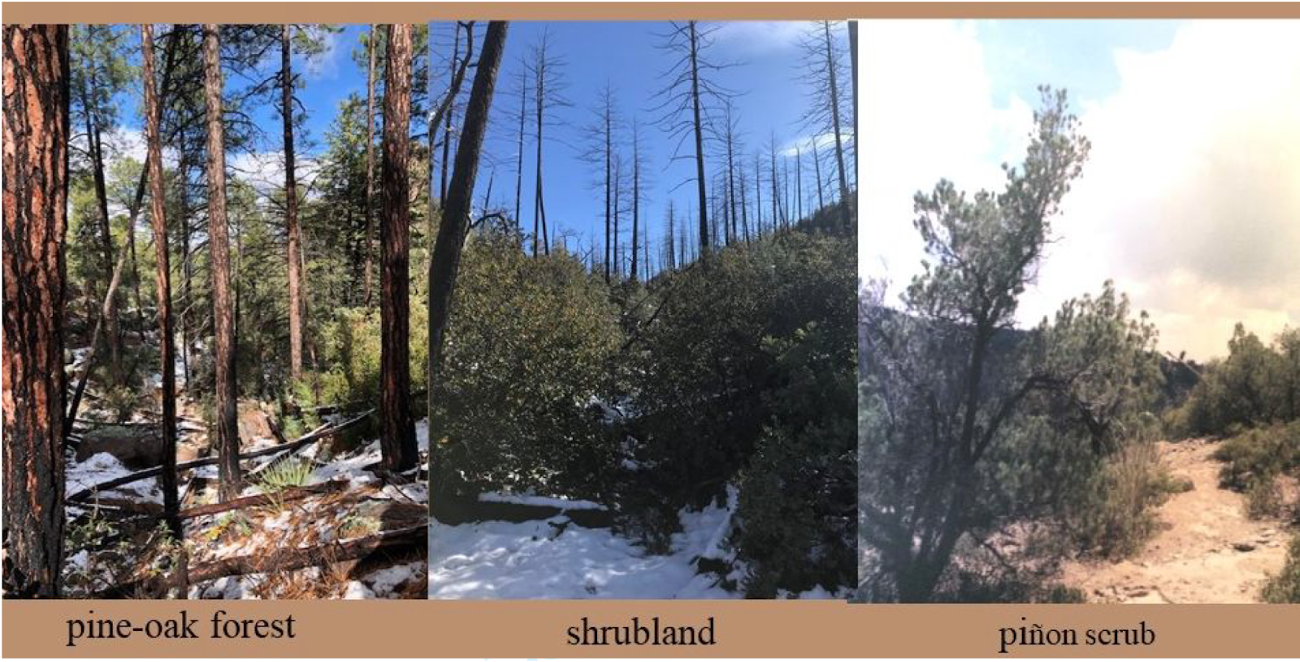The image contains a triptych of photographs, each bordered by brown lines, with the bottom line being more pronounced. The first photograph on the left, labeled "Pine Oak Forest," depicts a pine forest in the middle of winter with numerous tall, barren trees, some of which are fallen and lying on the ground. The central photograph is labeled "Shrublands" and shows a winter scene with green shrubs thriving amidst the snowy ground. In the background of this photo, barren trees can also be seen in the distance. The final photograph on the right, labeled "Pinon Scrub," displays a landscape that appears to be a desert environment, possibly photographed during the summer, featuring sandy soil with various desert plants growing on both sides of the image. Each photograph distinctly portrays different types of ecosystems, emphasizing the contrast between the seasons and vegetation within these landscapes.